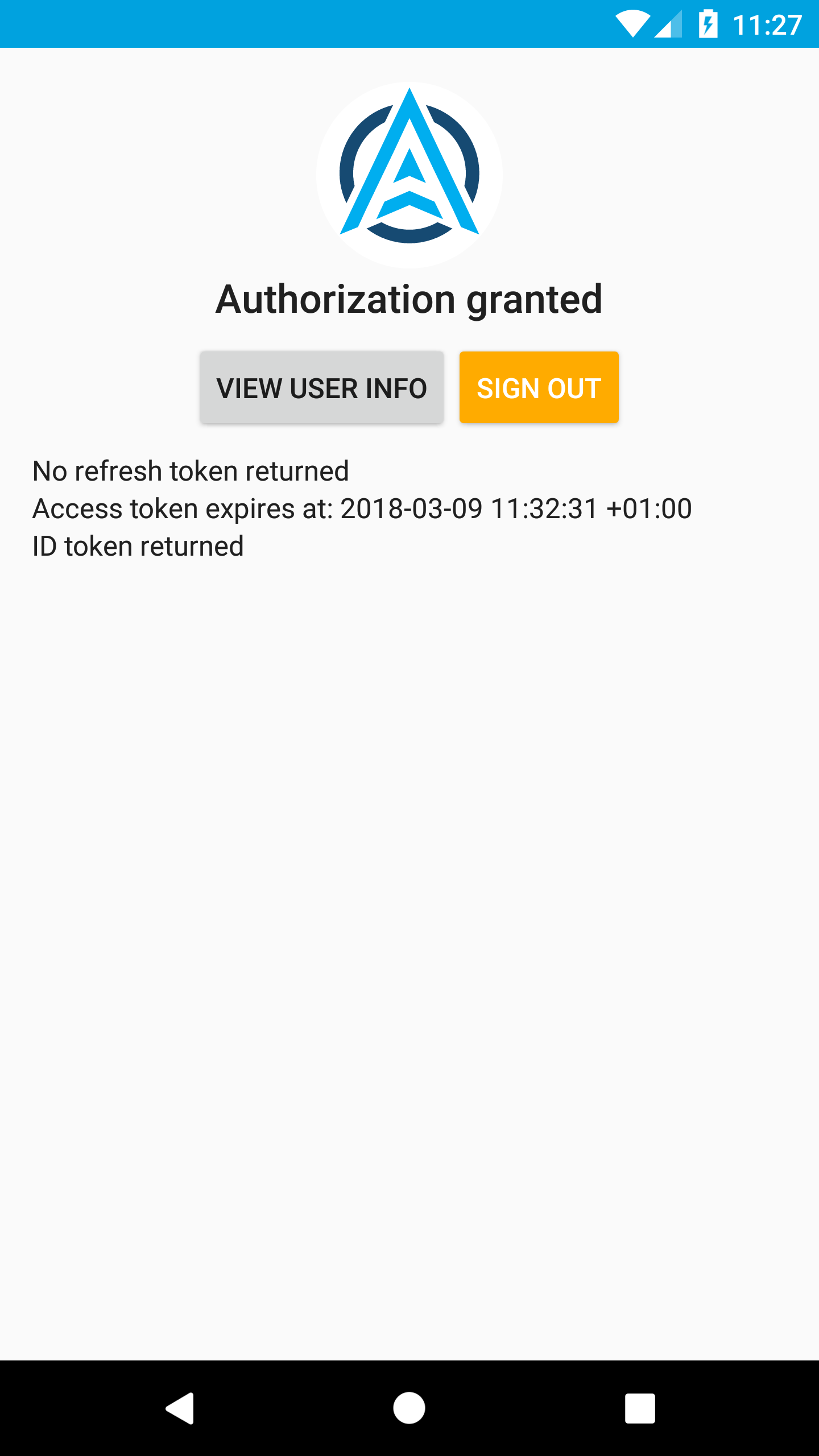The image depicts a cell phone screen with a blue border at the top. In the top right corner, icons representing wireless signal strength, cellular connection, and a charging battery are displayed next to the time, which reads "11:27." 

Centered below this is a prominent graphic of a stylized letter "A" intersecting a broken circle, which is divided into three parts. The circle is a deep purple or dark blue, while the "A" is a lighter blue. Below this graphic, the text "Authorization Granted" is clearly visible.

Two buttons are situated directly below this text. The first button, with a gray background, is labeled "View User Info." Next to it, a button with an orange background and white text reads "Sign Out."

Further down the screen, a line of text reads: "No refresh token returned. Access token expires at 2018-03-09, 11:32:31 +01:00. ID token returned." The remaining portion of the page has a light gray background without any additional text, images, photos, or drawings.

At the bottom of the page, a black border spans the width of the screen, containing three distinct white icons: a left-pointing arrow on the left, a small circle in the center, and a square on the right.